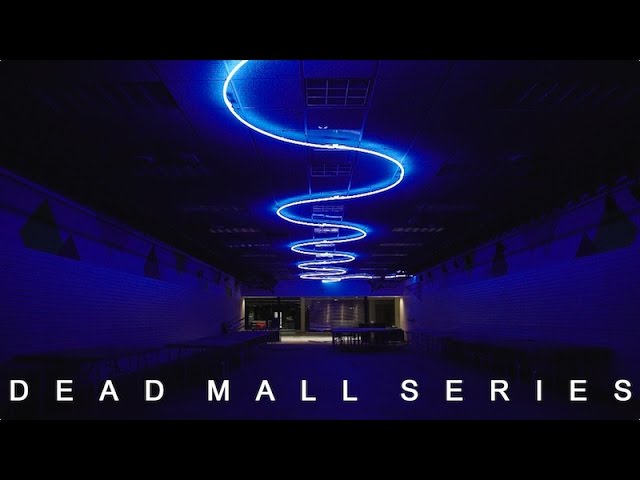The image is a detailed and atmospheric advertisement for the "Dead Mall Series," a show presumably by YouTuber Dan Bell. It showcases an expansive, dimly lit room within an abandoned mall. The primary source of illumination is a squiggly, neon blue rope light that weaves across the ceiling, casting a faint, eerie glow throughout the space. The room is depicted with a dead-on perspective, enhancing the sense of depth and emptiness. On either side of the room are unused tables and bare white walls, suggesting former commercial use. To the far end, the room opens into a pathway that leads to more vacant areas, hinting at additional desolate spaces for small businesses. The predominant colors in the image are blues and blacks, contributing to the overall haunting and somber mood. At the bottom of the image, white text reads "Dead Mall Series," firmly anchoring the theme of the visual.